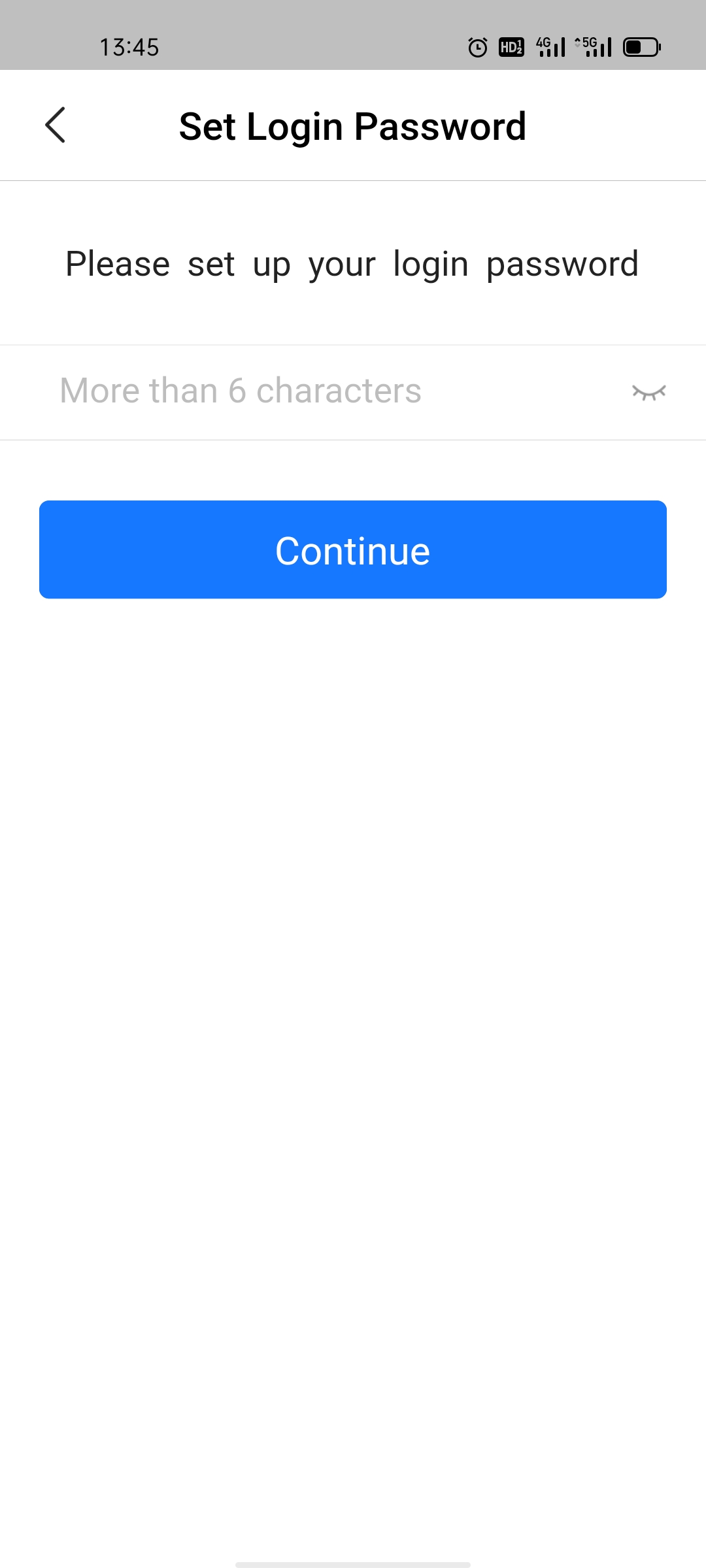Screenshot Description:

The screenshot captures a section of a smartphone screen taken at 13:45. At the top of the screen, common status indicators are visible: an active alarm, both HD 1-2 icons, 4G and 5G signal strengths, and a battery icon showing approximately 50% charge. The main content displays a minimalistic interface for setting a login password. Against a white background, the heading "Set Login Password" is prominently written in a black font. To the left of this heading is a left-pointing arrow, suggesting a navigation option to return to the previous page.

Below the heading, the phrase "Please set up your login password" is displayed, providing further instruction. In the input field for the password, a placeholder text in gray reads, “Password must be more than six characters long.” Adjacent to the input field, a closed-eye icon with eyelashes indicates that the password is currently hidden, and can be made visible if the icon is tapped. At the bottom of the page, a blue button labeled "Continue" in white text allows the user to proceed once a password is entered. The page is otherwise unadorned, emphasizing simplicity and clarity in its design.